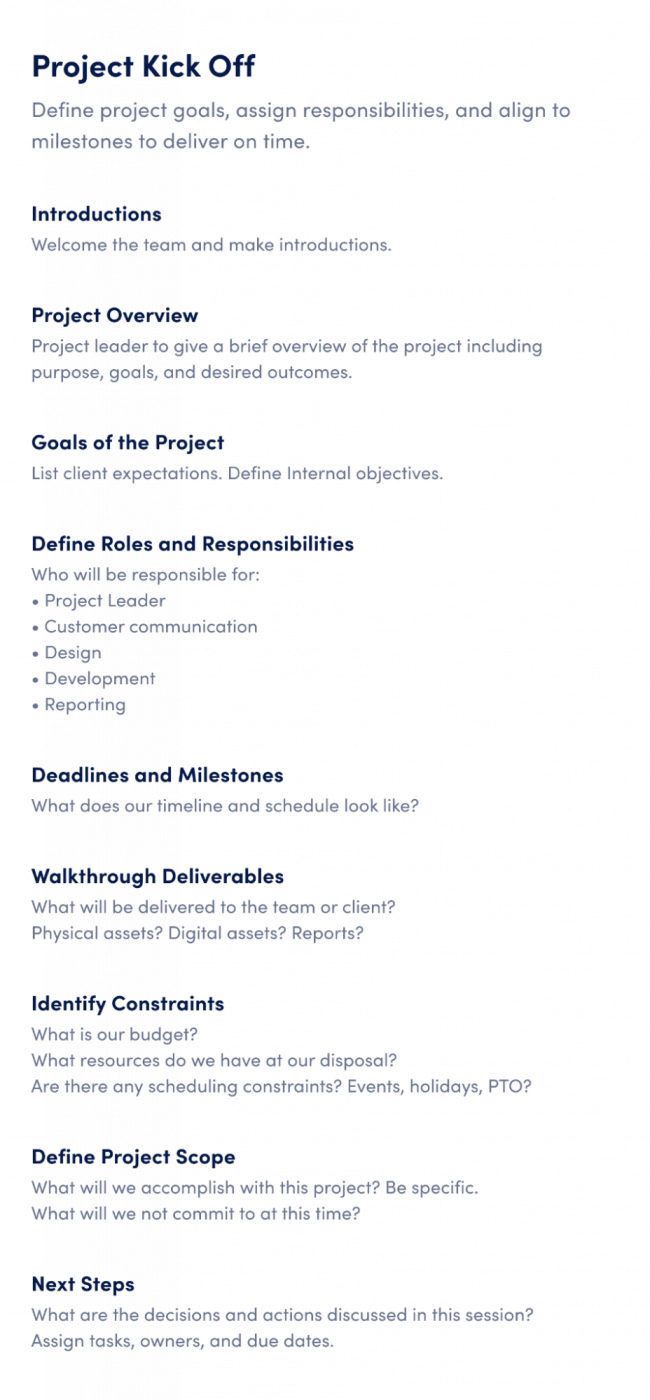**Caption:**

On a white background, the image displays a structured vertical list of information, primarily in navy blue and gray text. At the very top, in bold navy blue text, it reads "Project Kickoff." Below this heading, in small gray text, the instructions are laid out: "Define project goals, assign responsibilities, and align to milestones to deliver on time."

The next section, titled "Introductions" in navy blue text, is followed by gray text that says: "Welcome the team and make introductions." 

Following that, the "Project Overview" section in bold navy blue text contains gray subtext indicating: "Project leader to give a brief overview of the project, including purpose, goals, and desired outcomes."

Subsequently, under the bold navy blue title "Goals of the Project," the gray text outlines: "List client expectations, define internal objectives."

The section labeled "Define Roles and Responsibilities" in bold navy blue text is followed by gray text stating: "Who will be responsible for: Project leader, customer communication, design, development, and reporting."

Finally, under the heading "Deadlines and Milestones" in bold navy blue, the gray text asks: "What does our timeline and schedule look like?"

The structured layout continues iterating down the page in this style, maintaining clarity and organization throughout.